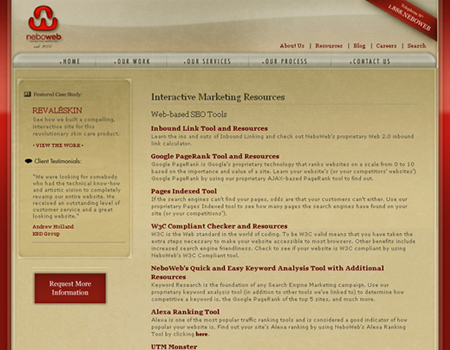This is a detailed screenshot from the Nebo website, featuring an "Interactive Marketing Resources" section. The image has a tan-colored background and includes a white sub bar stretching across the top, which contains unreadable menu options. On the left side, there is a vertical toolbar with additional unreadable menu items. The central heading, "Interactive Marketing Resources," is clearly visible, followed by a list of seven options, each in red text. Unfortunately, the subtext beneath these options is too small to distinguish.